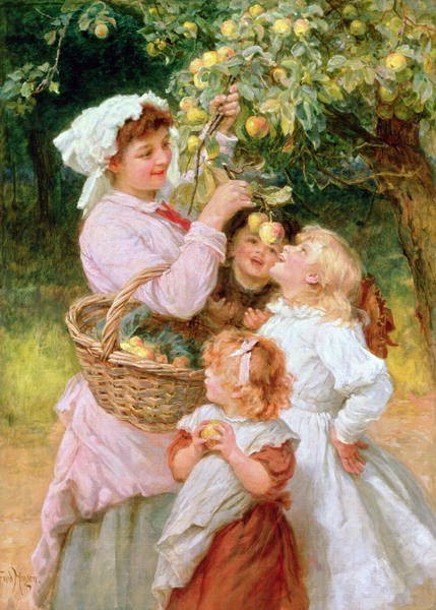In this 19th-century-style painting, a woman dressed in a pink dress, adorned with a white bonnet and a red bow near her collar, is depicted in an orchard with three young girls. The woman is standing beneath an apple tree, holding a woven basket over her right arm, filled with orange-yellow apples and green leaves. With her right hand, she reaches up to pluck more apples from a branch, which she pulls down with her left hand to make them accessible. 

The three girls, who appear to range from four to seven years old, are gathered around her, each uniquely characterized by their attire and actions. One girl, with red or light brown hair tied with a pink bow, is dressed in a reddish-brown dress with a bib-like garment around her neck and clutches an apple as she gazes into the basket. Another girl, sporting blonde hair and a pure white dress, looks up at the woman with a smile, seemingly excited about the apples. The third girl, standing slightly behind, has dark hair and a more ambiguous appearance, with her face partly obscured by the apples she is admiring. 

The background reveals a serene forest setting, adding a natural and wholesome ambiance to the scene, as the group shares a moment of joy and togetherness amidst the apple trees.